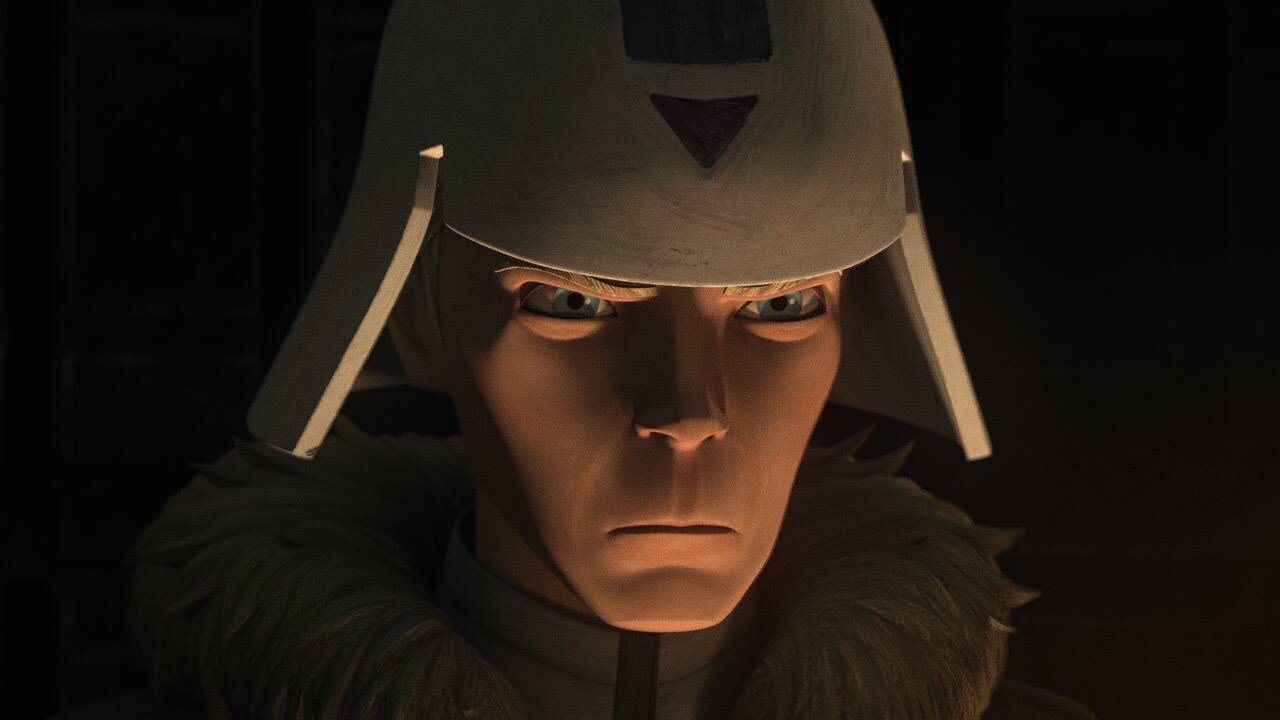In this image set against a stark black background, a man with a noticeably angry expression is depicted in what appears to be digital video game graphics, exhibiting a 3D clay-like effect. He is centrally positioned, illuminated from below which accentuates his menacing demeanor. His face is tan with blue eyes that are set wide apart, characterized by a scrunched expression and tightly pressed lips forming a straight line.

The man is wearing a distinctive grayish helmet reminiscent of a stormtrooper's, featuring two rectangular flaps extending down over his ears. On the helmet, there's an upside-down brown triangle and a small brown rectangular piece at the top. His attire includes a fur-collared jacket, likely brown, with a texture that somewhat imitates feathers projecting outward. The jacket appears to have a central black line, possibly a zipper, suggesting it might also serve as a fur-trimmed turtleneck sweater with a zippered closure. The overall scene provides a dark and foreboding atmosphere, with the character giving a piercing, almost deathly stare.